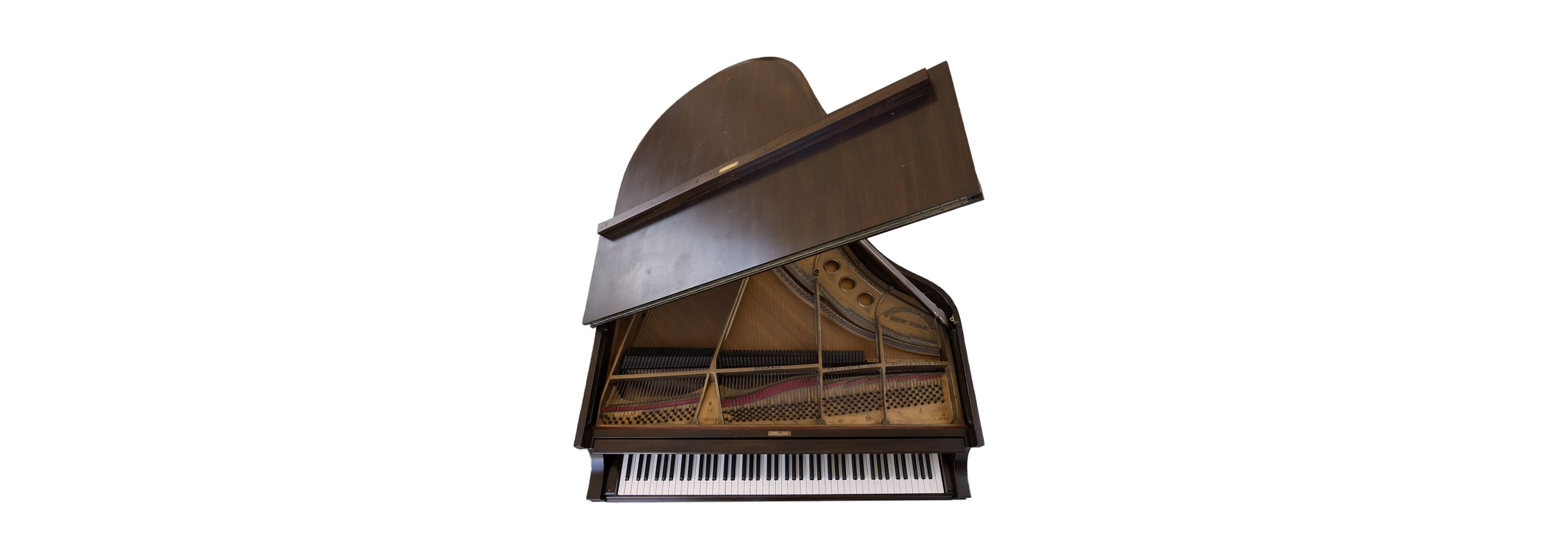The image showcases a grand piano set against a white background, viewed from a top-down perspective. The piano features a chocolate brown exterior with a raised lid, revealing a light brown interior. Its keyboard consists of black and white keys, arranged with black separators between the white keys. The top portion of the piano slopes upward and curls slightly to the right. This detailed depiction includes the flat rectangular lid area and visible grayish strings inside the instrument. Notably, the piano's legs are not visible in the photograph, emphasizing the keyboard and upper section of the piano. No one is currently playing the piano.